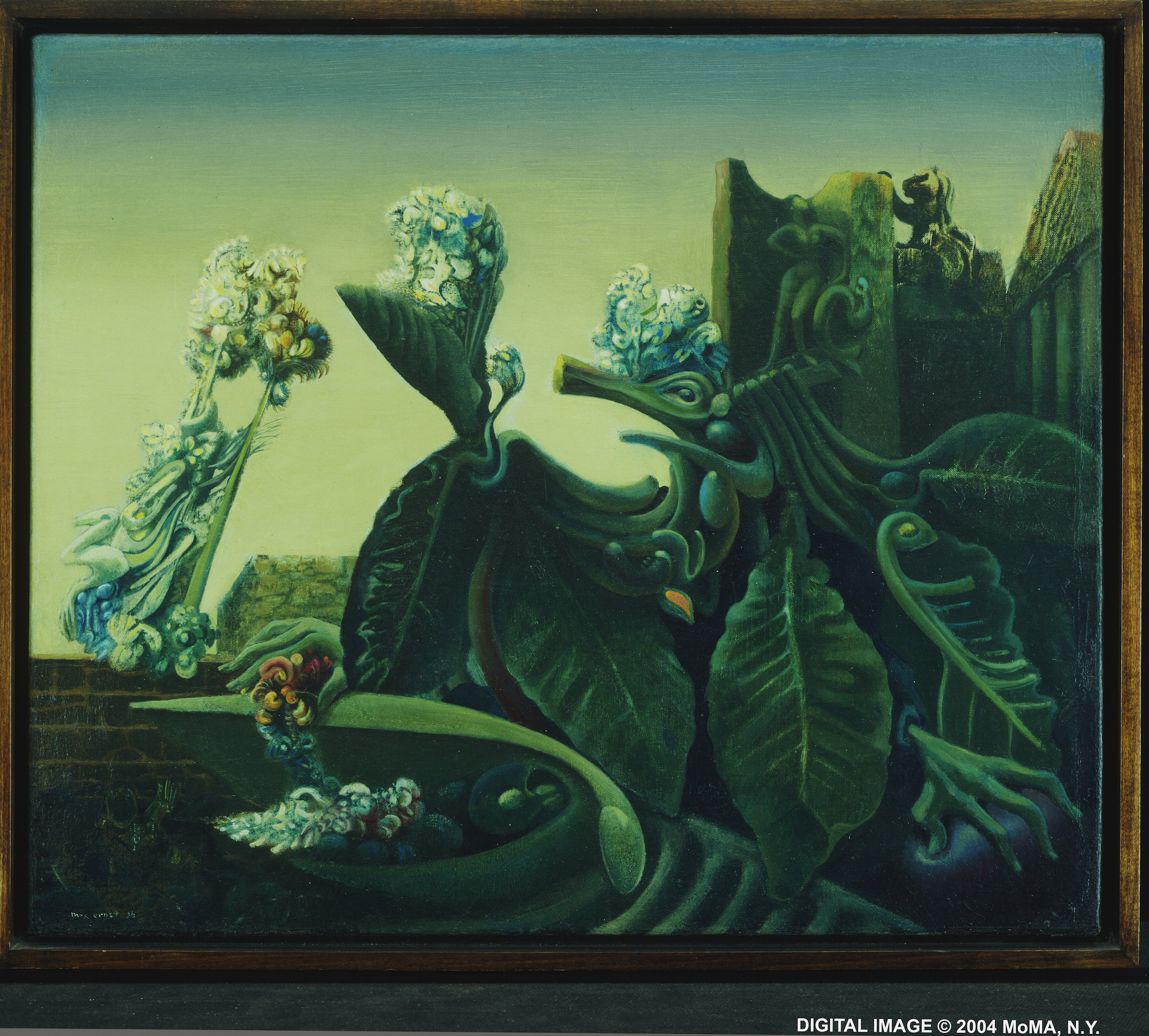The image showcases a cluster of dark green leaves, each intricately detailed with prominent veins running along their sides. The leaves are attached to coiled stems, adding a sense of natural elegance to the composition. Atop these lush, life-sized leaves, delicate flower petals are visible, contributing to the scene's vibrant beauty. Surrounding the main foliage, small green statuettes of people pepper the background, creating a whimsical and artistic touch. The scene is set against a serene, light blue sky, completing the picturesque and tranquil atmosphere.